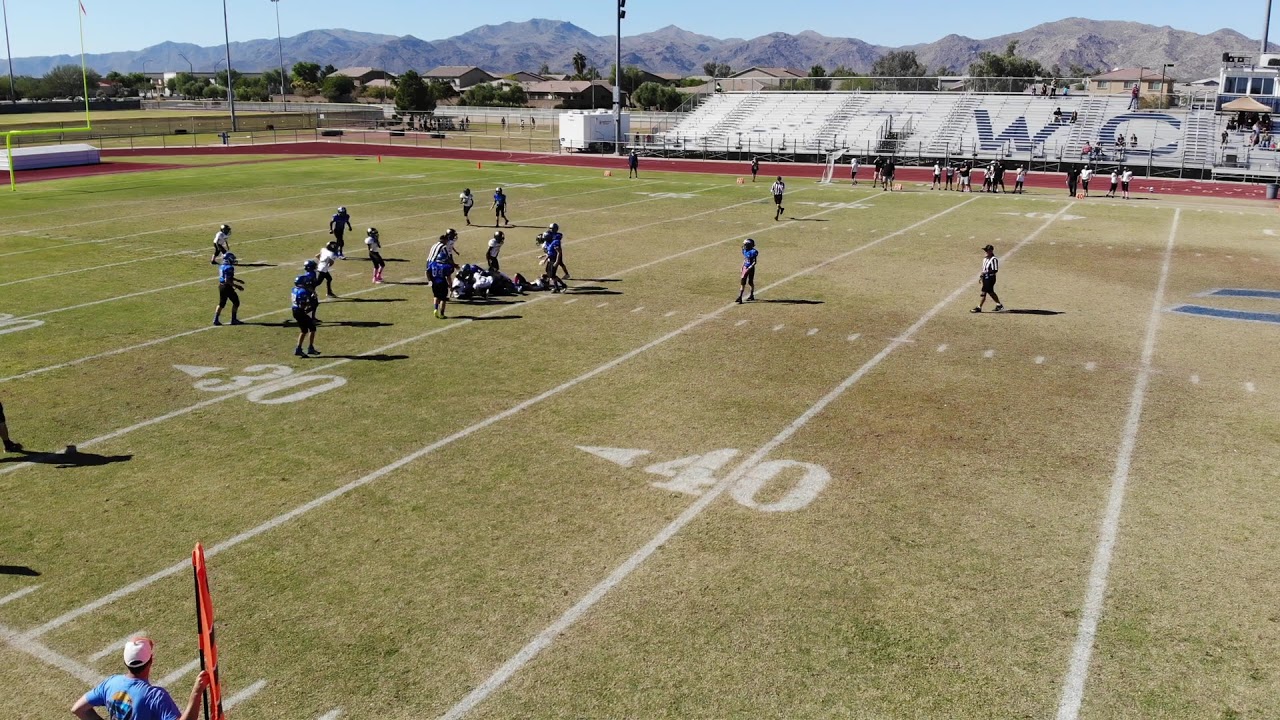The image captures an active football field, primarily focused around the 40 and 30-yard lines. The turf varies in vibrancy, with sections of lush green grass contrasting against dry, brown patches. Players are distributed across the field, some standing, others seemingly in the midst of play, wearing blue and white jerseys. Near the 40-yard line, a referee stands poised while another one is in motion coming down from the 30-yard line. 

To the right, the bleachers bear the large letters "WC," and are sparsely populated. A small shed and additional structure are positioned nearby. The stands have white posts and feature a noticeable bench with the letters "W" and "O." In the far backdrop, a range of rocky, brown hills accentuates the clear blue sky. Nearby the players, a person in a blue shirt and white hat holding a yellow object, likely a line judge, is visible on the bottom left. A first down marker is also observable in the bottom left corner.

In the middle of the scene, two players stand near the 40-yard line while a cluster gathers around the 30-yard line, suggesting a possible tackle. The field markings are clear, with large white numbers denoting the 40, 30, and 20-yard lines, and horizontal lines marked every five yards, interspersed with smaller rectangles indicating individual yards. A dark blue logo appears faintly on the furthest right side of the image.